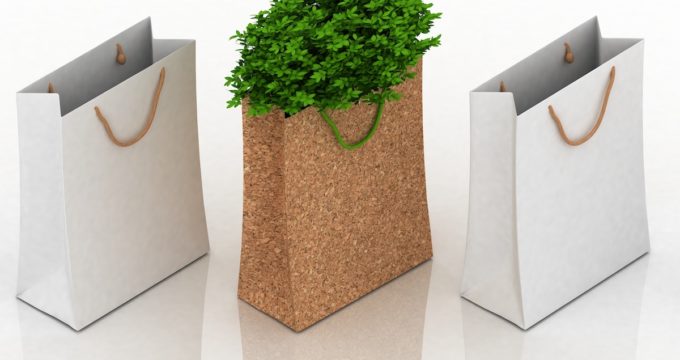In the image, three gift bags are neatly aligned on a glossy white table, their reflections slightly visible due to the table's sheen. The two bags on the left and right are identical, pristine white with light beige rope handles, securely attached and oriented towards the lower right corner of the image. The bag in the middle, which captures the most attention, is distinct with its sandy, gravelly texture resembling tack board material. This middle bag boasts a vibrant green handle that matches the striking foliage spilling out from its top, injecting a burst of greenery into the scene. The contrast between the simple, empty white bags and the plant-filled, textured middle bag creates a captivating visual dynamic, with the central bag's rich, earthy tones and lively greens drawing the viewer’s eye.